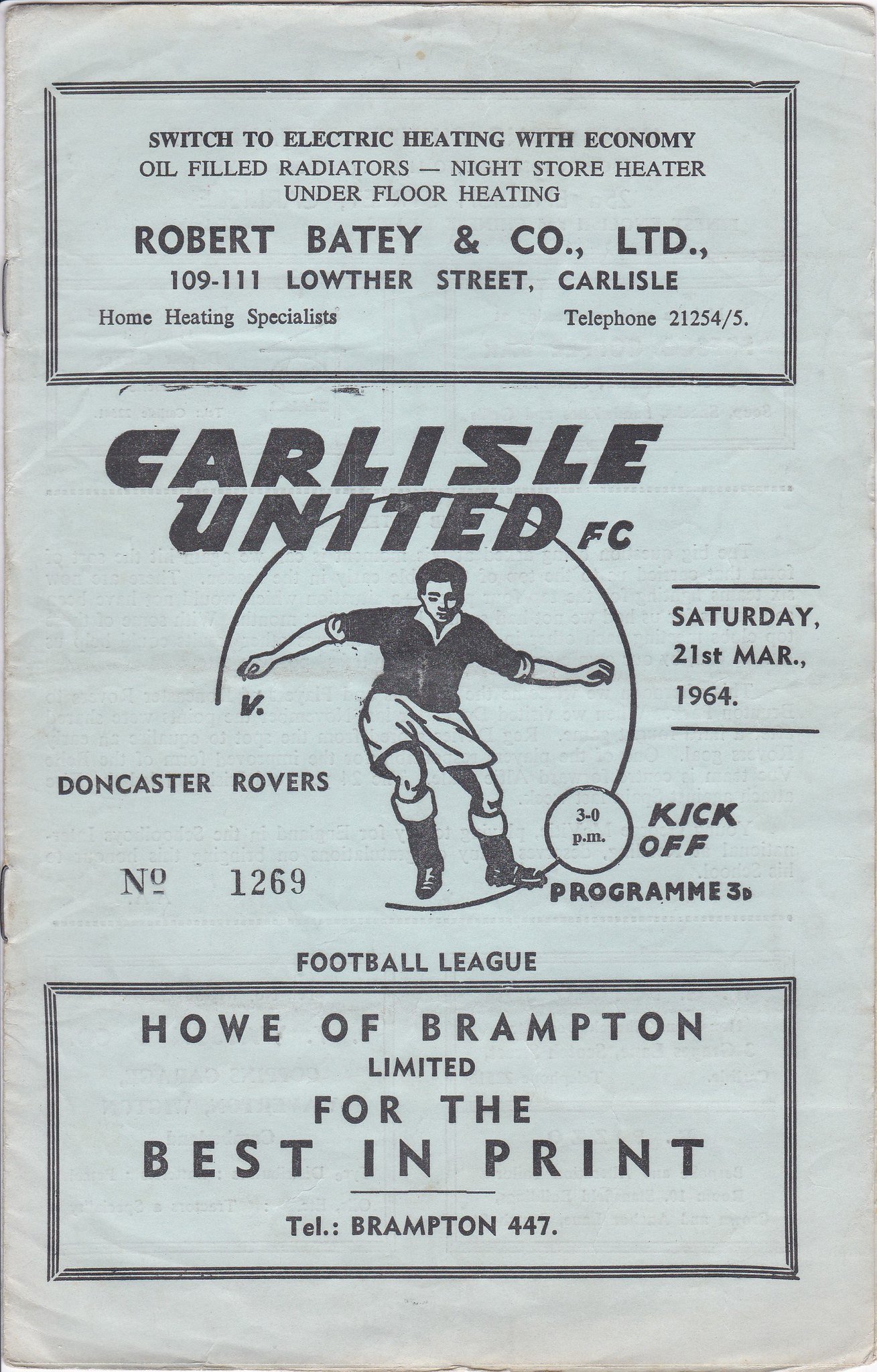This image appears to be an old, slightly wrinkled, black-and-white advertisement, possibly from a magazine or newspaper. The corners of the paper show signs of being folded and there are two staples on the left, indicating it was once part of a bound collection. The top of the advertisement features a black-lined bordered rectangle containing text that reads: "Switch to electric heating with economy. Oil-filled radiators, night store heater, underfloor heating. Robert Beatty & Co. Ltd, 109-111 Lowther Street, Carlisle. Home heating specialists. Telephone number: 21254-5." 

In the center of the image, there's an illustration of a young boy in soccer attire, suggesting he's playing the sport. Above this illustration, in bold, it reads "Carlisle United FC." Additional text around the graphic mentions "Doncaster Rovers, number 1269, Saturday 1964 kickoff program." At the bottom of the advertisement, another promotion reads, "Howe of Brampton Ltd. for the best in print. Telephone Brampton 447."